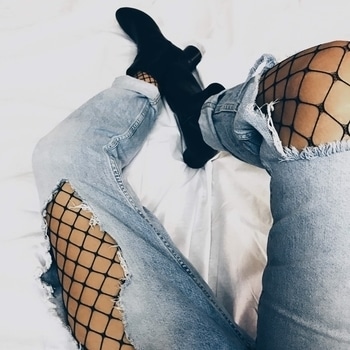The image captures a top-down view of a woman’s legs in a relaxed pose, presumably lying on a solid white sheet or bed. She is wearing light, distressed denim jeans with significant rips; the left leg features a large tear above the knee extending over most of the thigh, while the right leg has a big hole at the knee. Underneath the jeans, she is wearing wide-weave fishnet stockings, revealing a peach-colored flesh tone through the rips. Her jeans are worn and faded, with the cuffs noticeably rolled up. She completes the edgy look with black ankle booties that have small heels and zippered sides. Her legs are casually crossed at the ankles, with the right leg bent slightly upward and the left leg resting straight. The photo distinctly shows only the area from her upper thighs, just below the crotch, down to her feet, emphasizing the stylish contrast between the torn jeans, fishnet tights, and black boots.